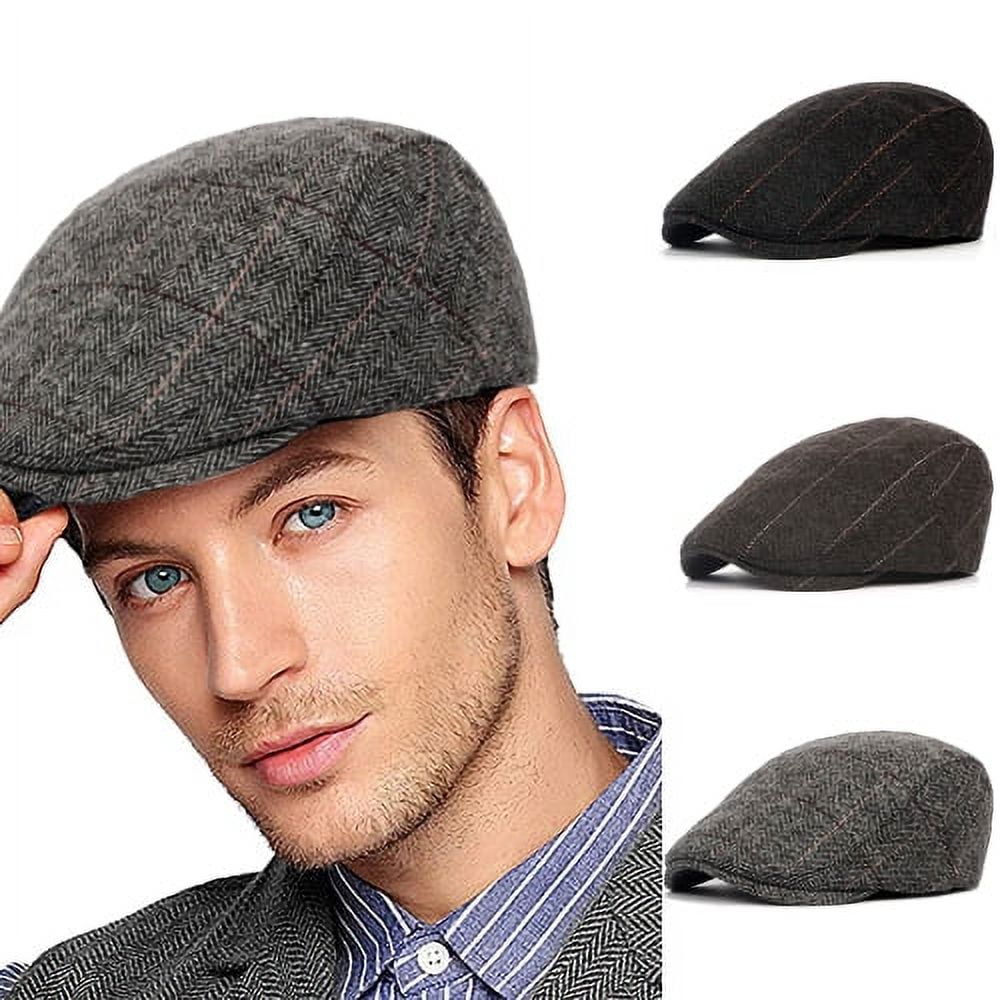This promotional photograph showcases a flat cap style hat, ideal for an e-commerce or product manufacturer website. Dominating the left side of the image is a handsome male model with blue eyes and a low trimmed beard, wearing a gray flat cap. He is dressed in a blue and white striped button-down shirt with a textured gray jacket, matching the material of the cap. His head is slightly tipped forward as he gazes into the camera. To the right of the model, three additional flat caps are presented against a pure white background, each in a slightly different color: a predominantly black one with faint pinkish stripes, a dark gray one with faint white stripes, and a gray one featuring faint pink stripes similar to the cap the model is wearing. The clean, white background emphasizes the hats, making this image ideal for showcasing product details and appealing to potential buyers.